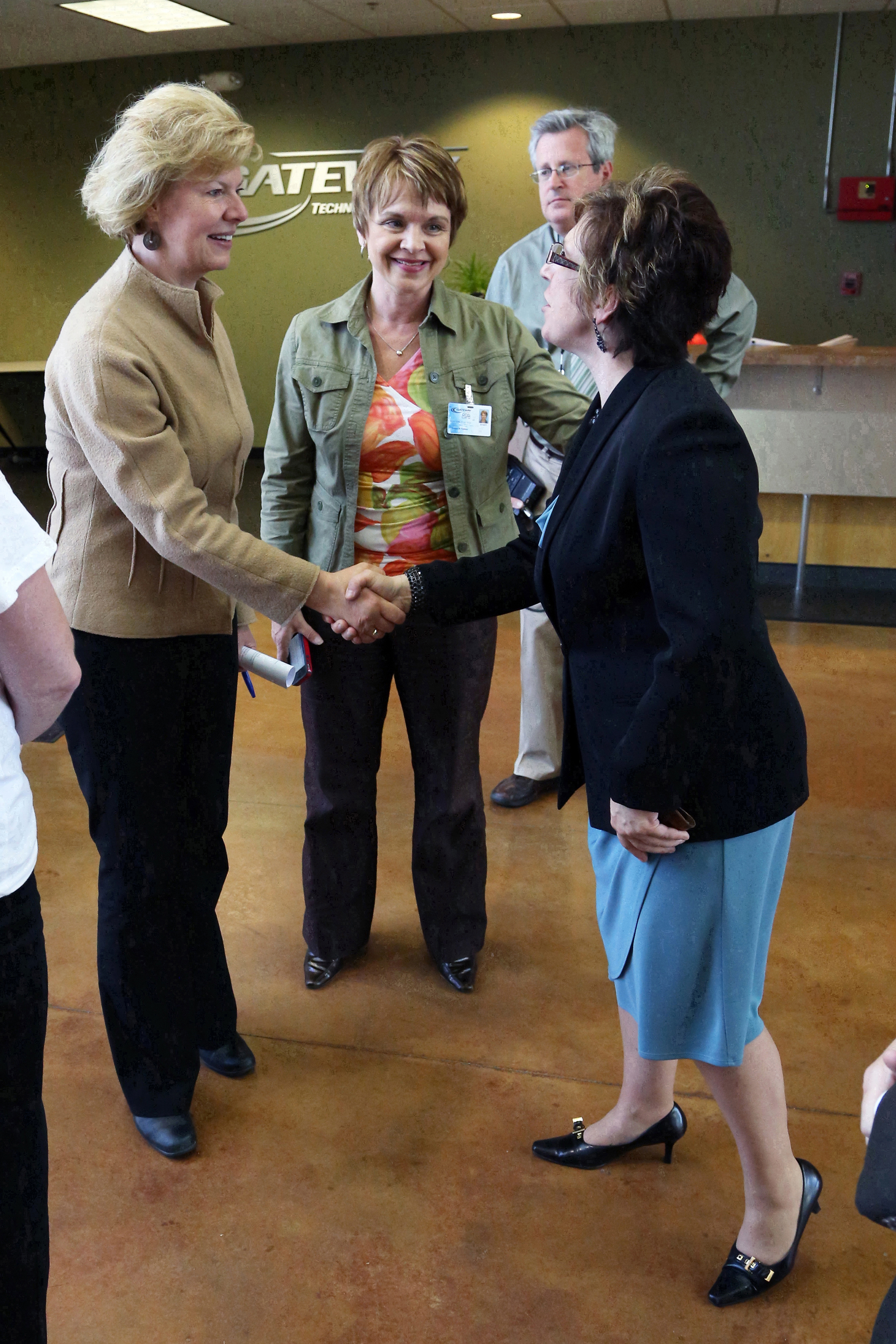In an interior photograph taken inside a large reception or meeting room with a grid-style white ceiling illuminated by fluorescent lights, three middle-aged women are engaged in a cheerful interaction, possibly at a conference or meeting. The room features a brown concrete floor and an olive-green wall in the background with a partially obscured logo related to technology. On the right, a woman with short brown hair, glasses, and a black blazer paired with a light blue skirt is smiling and shaking hands with another woman to her left. This woman has blonde, ear-length hair and is dressed in a tan jacket, black slacks, and black shoes. Standing between them and slightly behind, another woman with light brown hair and a colorful floral blouse in orange, pink, and green under an olive green jacket extends her hand towards the woman in the blue skirt, seemingly congratulating her. She has a name tag clipped to her jacket. A gray-haired man with glasses, dressed in a blue shirt and tan slacks with brown shoes, stands slightly behind the women, observing the interaction with a congenial expression. Additional attendees are partially visible at the edges of the photograph; one woman on the far left is seen wearing a white shirt and black pants. The scene captures a moment of celebration and camaraderie among the participants.